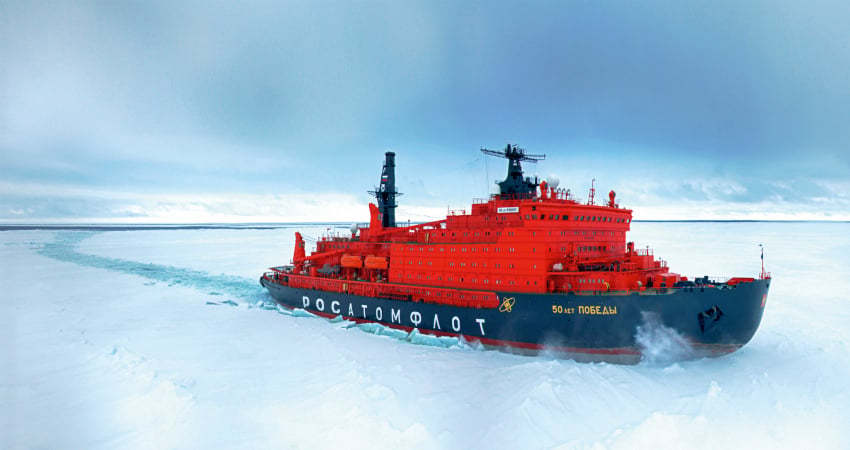This is a color photograph depicting a massive ocean vessel, likely an ocean liner, navigating through ice-covered waters in what appears to be an Arctic or similar cold region. The vessel has a prominent, dark blue hull and a vivid red upper structure housing multiple floors of cabins, which range from four stories at the rear to six stories at the front. Dominating the side of the hull is large, foreign text, possibly in Russian or German, featuring characters that resemble "P-O-C-A-T-O-M" with distinct symbols such as a slanted O with a line through it and an upside-down V. The ship is actively breaking through the ice, leaving a clear path of open water in its wake. The ice surrounding the vessel is a striking combination of white and blue, contrasting against the dark, stormy sky overhead. The top front of the vessel features large, square windows spanning the width, and the ship is equipped with various structures atop, contributing to its imposing appearance.